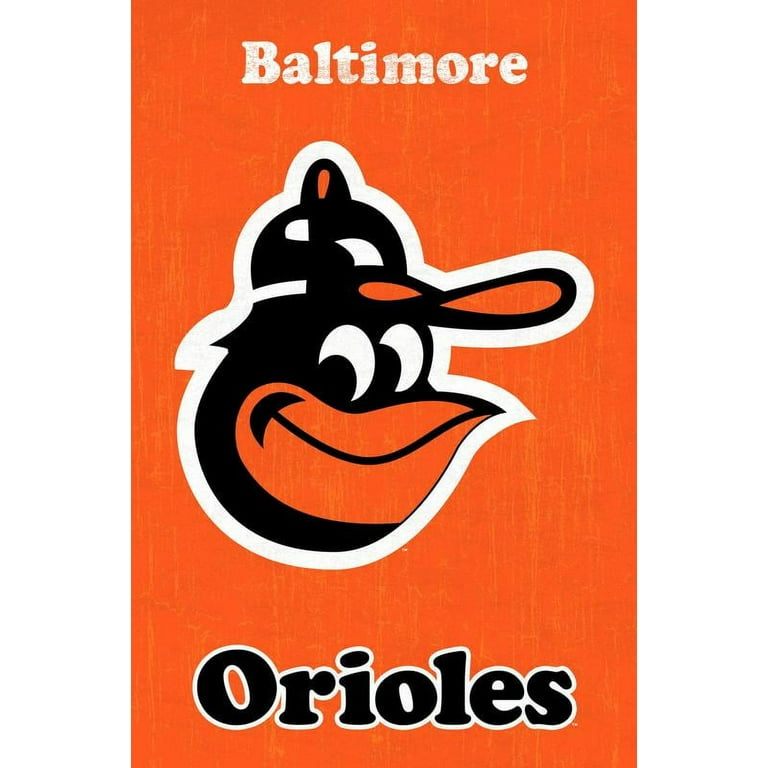The image displays a vintage-looking Baltimore Orioles sports poster with a weathered appearance, featuring a bright orange background. At the top, "Baltimore" is written in white letters, subtly streaked with orange. Centered in the middle is a cheerful cartoon bird, predominantly black with a white outline. The bird is wearing a black baseball cap with an orange bill and a small orange nub on top. Its beak is bright orange, matching the background. The bird's eyes are white, and it has a friendly smile. Below the bird, the word "Orioles" appears in black letters bordered in white, with both 'O's slanted—the first 'O' having an orange center and the second 'O' having a white center. The sign itself has a washed look, as if paint dripped during application, giving it a streaky, textured finish.